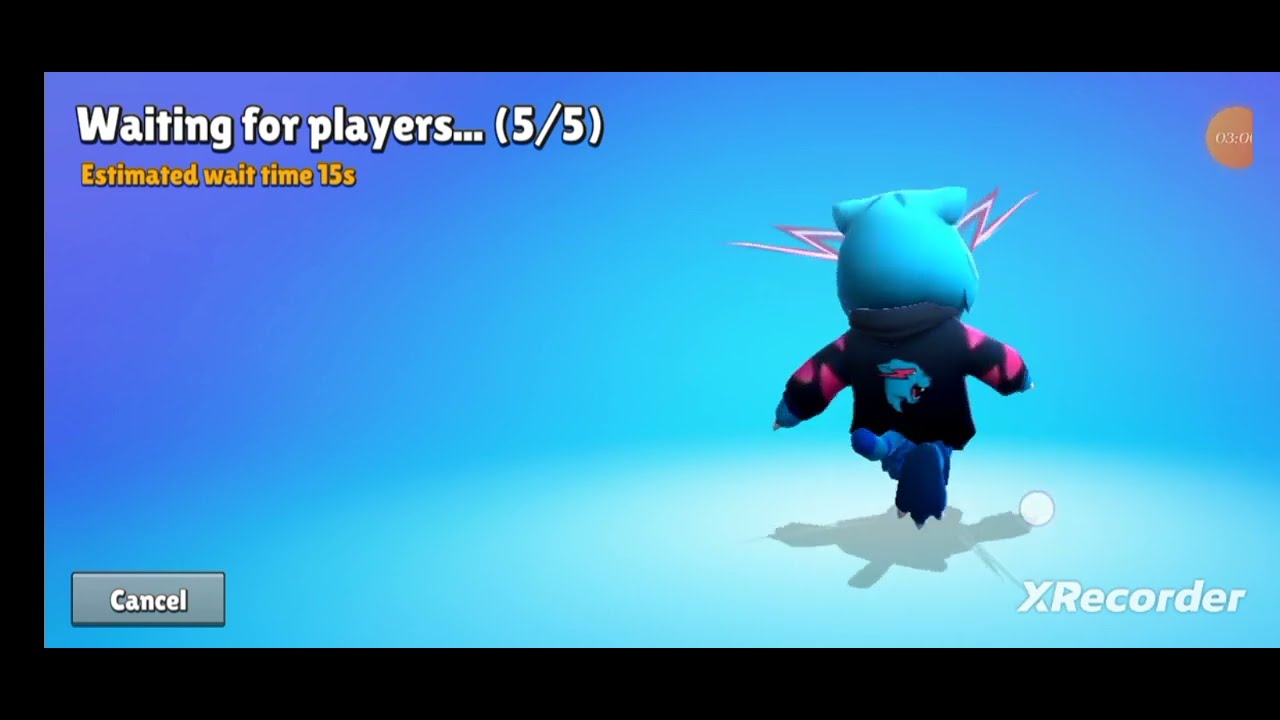The image is a screenshot from a video game, depicting a waiting screen. On the left side, a blue video game character stands out prominently. The character is outfitted in a black hoodie featuring a blue wolf graphic on the front, with pink stripes running along the sleeves. Pink antennas protrude from the sides of its head, while its feet are blue with three white, claw-like points. The character's simplified face shows minimal details—just eyes and a small mouth.

At the top left corner of the screen, white text reads "waiting for players... 5/5," and directly beneath it, yellow text states "estimated wait time: 15 seconds." In the bottom left corner, there is a gray cancel button. On the bottom right, the text "X recorder" appears in white. The entire scene is set against a light blue background.